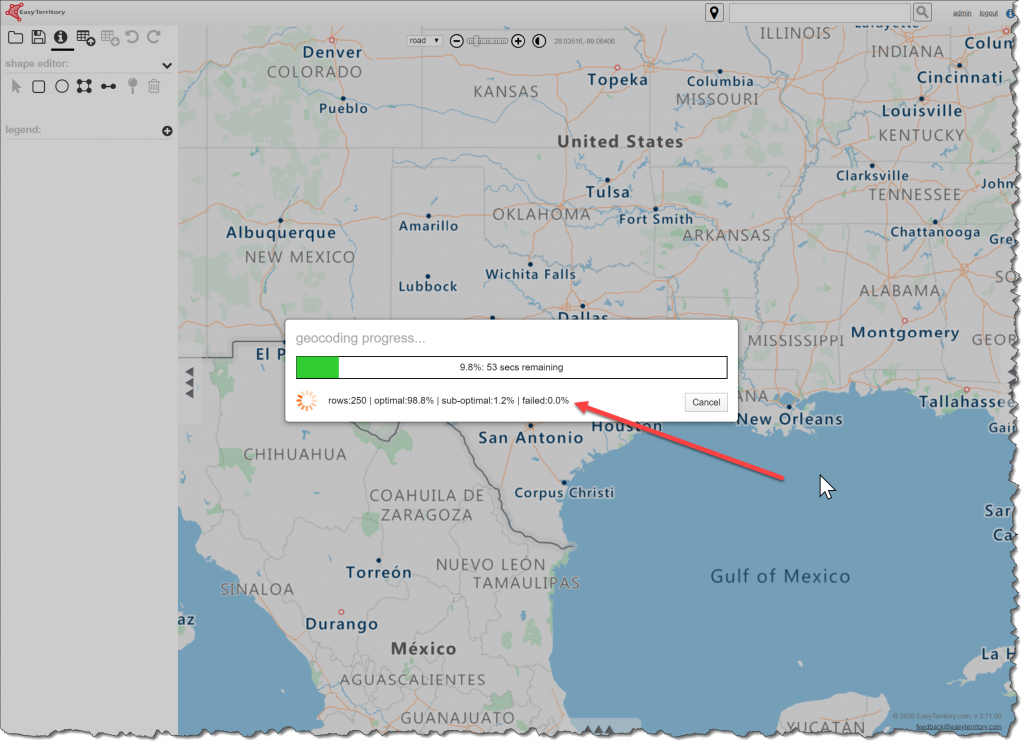This detailed image depicts a map of a section of the United States. The label "United States" is prominently written in dark font near the top-right quarter of the image. The upper left-hand corner features a small logo with a vertical column of icons beneath it, likely representing editing tools. The map displays several states in a gray all-capital letter font; notable states include Colorado, New Mexico, Kansas, Oklahoma, Arkansas, Missouri, Illinois, Indiana, Kentucky, Tennessee, Alabama, parts of Georgia, Mississippi, and Texas.

In Colorado, the cities of Denver and Pueblo are marked in blue font, while in New Mexico, Albuquerque is similarly highlighted. The map shows a jagged border on the right and bottom edges, contrasting with straight edges on the top and left sides. 

A white rectangular pop-up window is centered in the image, titled "Geocoding Progress" in light gray font. Inside, a section outlined in black contains a progress bar, partially filled in bright green, indicating 9.8 percent completion. Below the bar, it indicates 53 seconds remaining, though the black font beneath it is unreadable. In the bottom right corner of the pop-up, the word "Cancel" is visible, with an arrow pointing to the text under the progress bar, which also refers to the 53 seconds remaining. The area starts in the Gulf of Mexico and extends towards the progress bar.